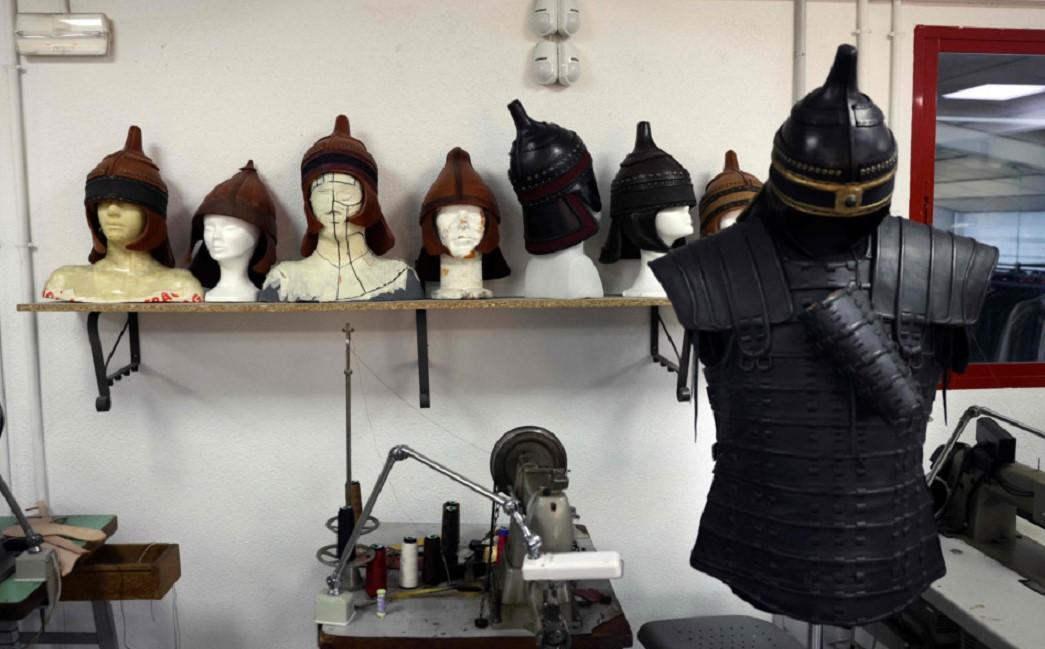The image is a detailed, color photograph in landscape orientation, showcasing the interior of a costume shop specializing in medieval-style armor and hats. Dominating the right side of the image is a suit of armor, displayed on an unseen mannequin, featuring an upper torso piece adorned with a black, pointed helmet accented by a gold band around the eye area. The armor, reminiscent of those seen in Japanese movies, includes a helmet with a plume, layered shoulder pads, and a leather-layered torso.

Behind this figure is a white wall adorned with a wooden shelf supported by metal brackets. The shelf holds approximately eight head mannequins, each adorned with various types of headgear. These include a mix of leather, fur, and steel helmets in different colors like black and brown. The arrangement shows four mannequins facing the viewer while the others are turned sideways, adding to the display’s dynamic appearance.

In the foreground at the bottom right, an industrial sewing machine indicates the craftsmanship involved in the shop, suggesting that the items on display are handmade on-site. A chair is positioned behind the sewing machine. To the left, partially cut off, is a work table. In the top right corner, a wooden-framed window with a red-bordered glass opening adds a pop of color, complementing the stylized realism of the photograph.